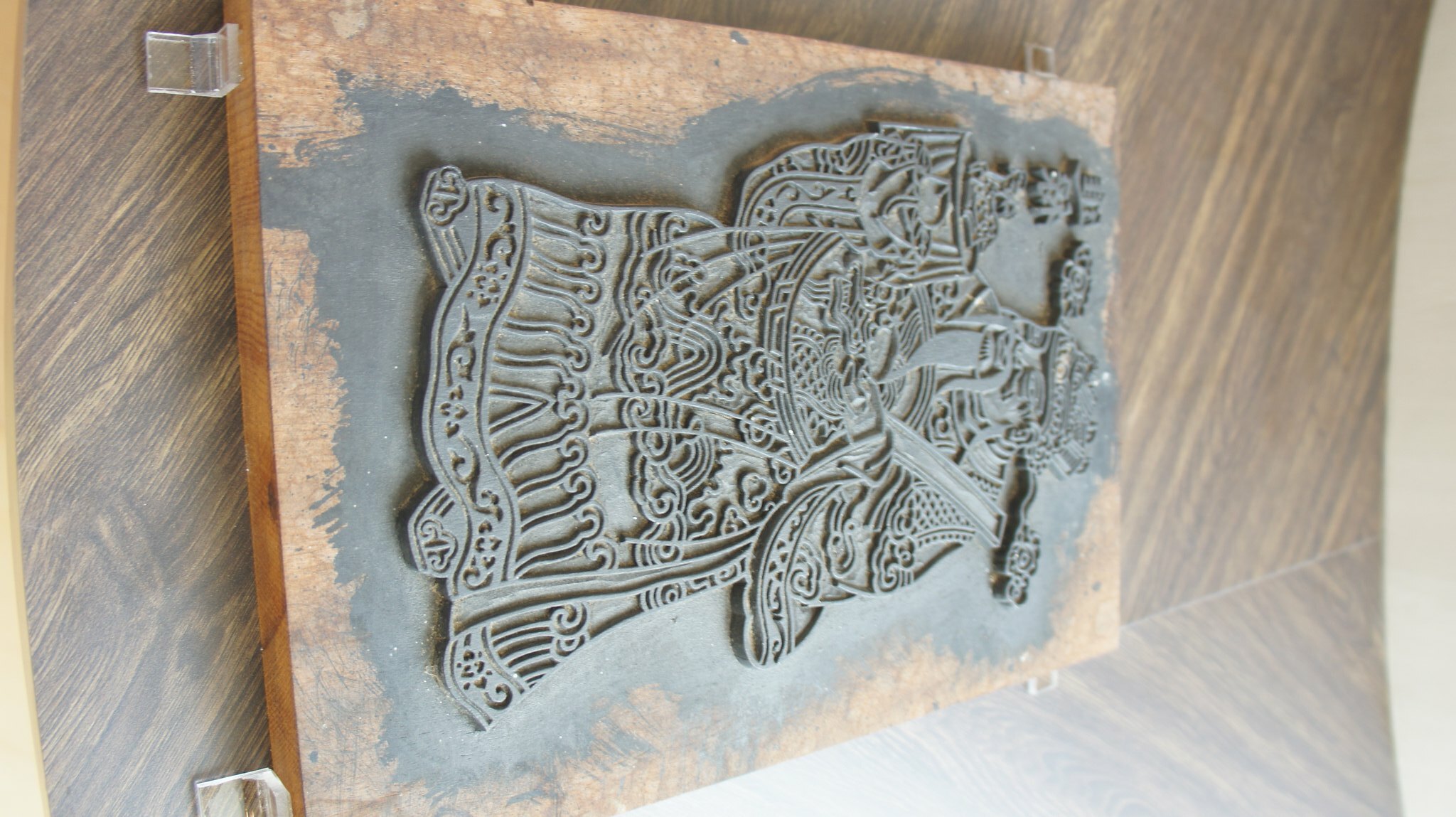This is an indoor, sideways photographic image depicting a wooden block used for printing. The block is mounted on a light brown table with a chevron grain pattern. The block consists of wood and a metal carving in bas-relief, featuring a detailed depiction of a Chinese man wearing traditional mandarin robes that flow down to his feet. The figure, who also sports a long mustache and beard, is holding an object, with Asian characters etched above him. The metal work on the wood block is gray, with some splotches of gray paint visible on the wooden surface. The block is attached to the white wall, and there are no texts in the image. The fine details and traditional attire suggest the figure could be interpreted as a notable Asian figure rather than a generic character.